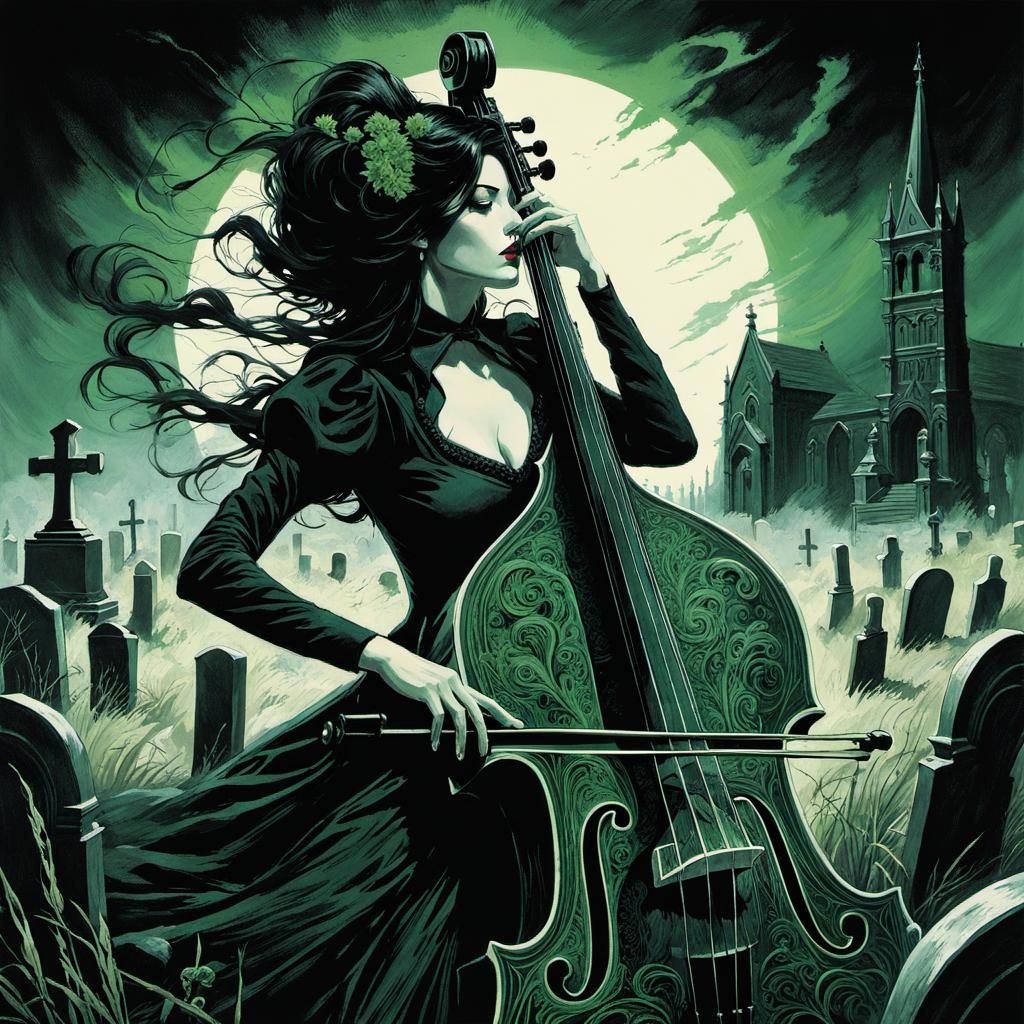In this captivating and intricate artistic interpretation, we see a stunning gothic cellist set against a hauntingly beautiful backdrop. The scene is dominated by a luminous full moon hanging low on the horizon, casting an eerie glow on the dark, cloudy sky. Wisps of haily green clouds float gracefully, enhancing the otherworldly atmosphere. A gothic church with a prominent steeple looms in the background, adding to the somber elegance of the setting.

In the foreground, a timeless cemetery with moss-covered tombstones and ancient markers creates a sense of history and reverence. The elegantly dressed cellist, embodying gothic aesthetics, commands attention with her ethereal presence. She is clad in a meticulously detailed black outfit that perfectly complements her long, flowing dark hair. Adorning her hair are delicate green flowers, adding a touch of nature to her otherwise dark ensemble.

Her cello, exquisitely designed, is an extension of her gothic elegance, resting gently in her hands. As she plays, the melancholic notes seem to resonate through the cemetery, creating a surreal and poignant scene. This masterful depiction captures the essence of gothic beauty, blending music, nature, and architecture into one mesmerizing image.